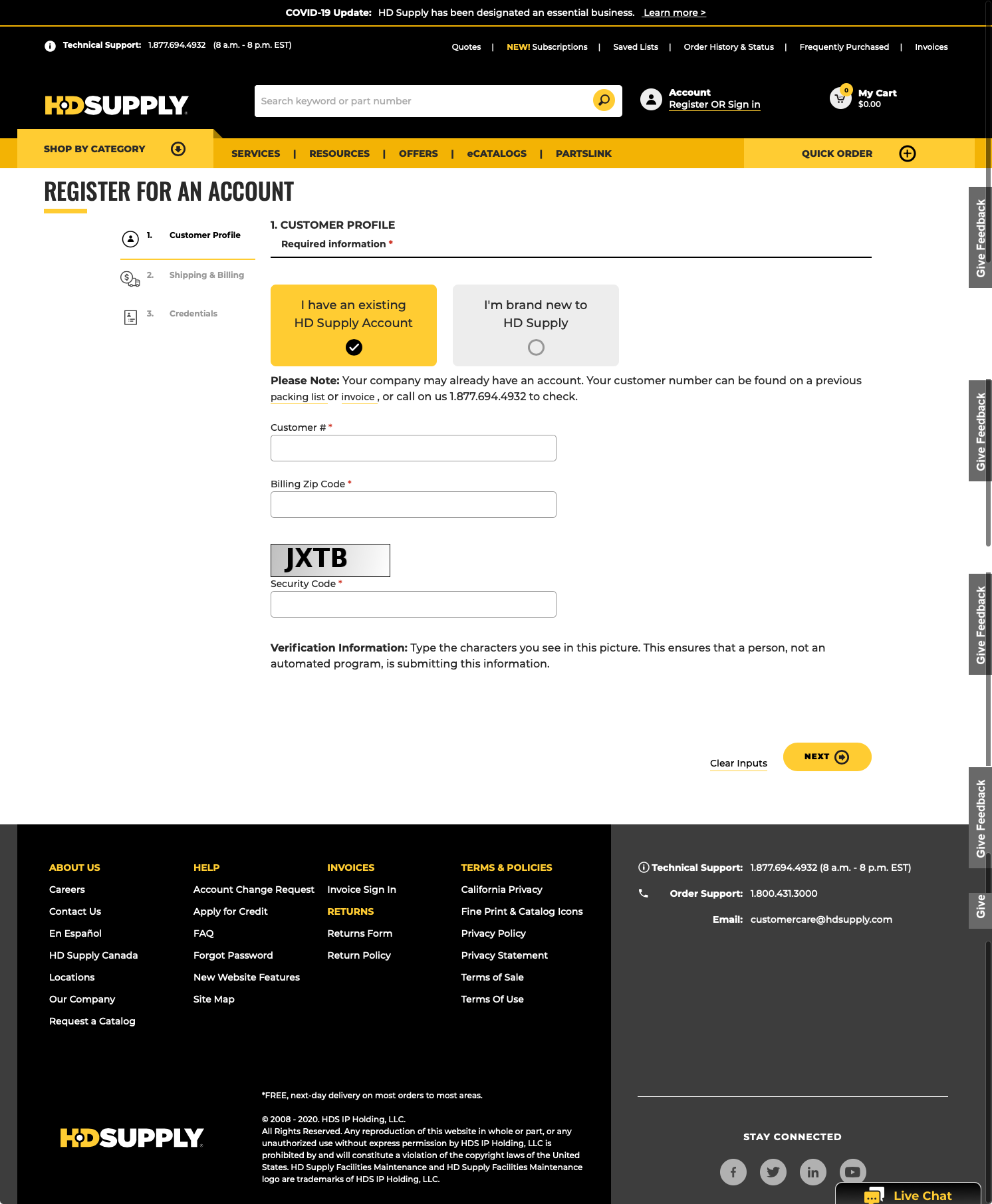The image appears to be a screenshot of a computer screen displaying the registration page of a website called "HD Supply." The site’s name, "HD Supply," is prominently displayed on a black header at the top, which also includes a search bar, options for "Account," and "My Cart."

The page has a white background in the main section, and the top black header houses navigation elements. The central portion of the page contains a title that reads "Register for an Account," followed by sections labeled "Customer Profile" and "Required Information."

There are two checkboxes, with the first one marked in yellow and checked, indicating, "I have an existing HD Supply account." The second checkbox remains unchecked and is labeled, "I'm brand new to HD Supply." A note beneath the checkboxes informs the user that their company may already have an account and provides instructions for locating their customer number on a previous packing slip or invoice, or by calling 1-877-686-6912.

Further down, there are fields for entering a "Customer Number," a "Billing Zip Code," and a pre-filled security code reading "JXTB."